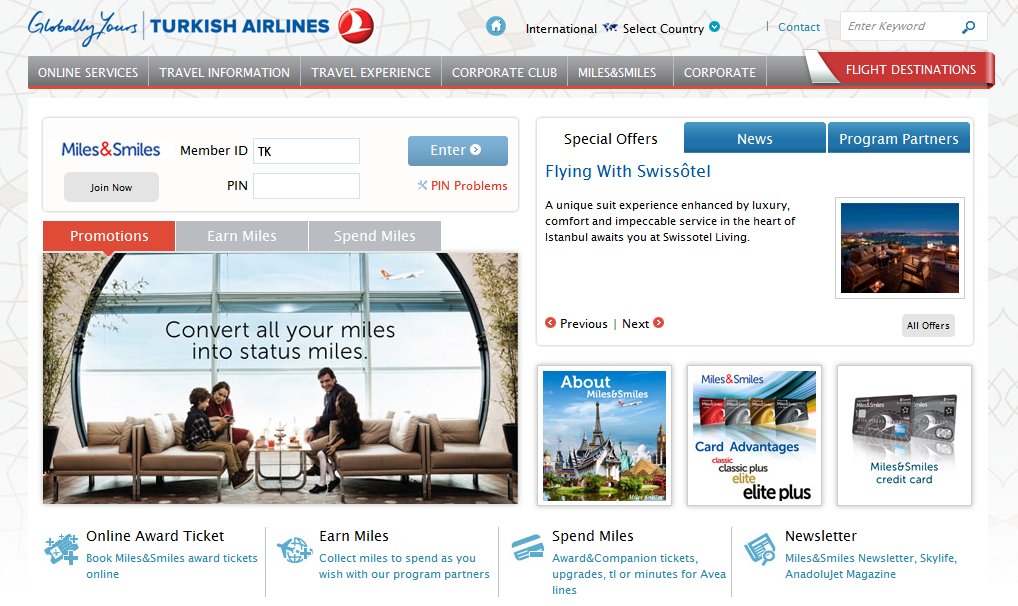This image features a Turkish Airlines webpage. Prominently displayed at the top is the Turkish Airlines logo, which consists of a white seagull in flight, enclosed within a red circle. Below the logo, there are navigation options that include 'Select Country,' 'International Contact,' and a search bar labeled 'Enter Keyword.' Beneath this navigation bar runs a horizontal gray line, within a rectangular section, containing further menu options: 'Online Services,' 'Travel Information,' 'Travel Experience,' 'Corporate Club,' 'Miles and Smiles,' and 'Corporate,' with 'Flight Destinations' highlighted in red.

Scrolling down, there is a section dedicated to the 'Miles and Smiles' loyalty program. Here, the text 'Join Now' invites new members, accompanied by a blue button for entering the program once you input your member ID and PIN. Additionally, there's a clickable 'PIN Problems' link in red for users experiencing issues.

Adjacent to this section, more options include 'Promotions,' 'Earn Miles,' and 'Spend Miles,' as well as a 'Special Offers' area featuring news about program partners like Swissotel. Visual elements include images showcasing various travel destinations and advertisements, providing an enticing glimpse into the wide array of locations Turkish Airlines serves.